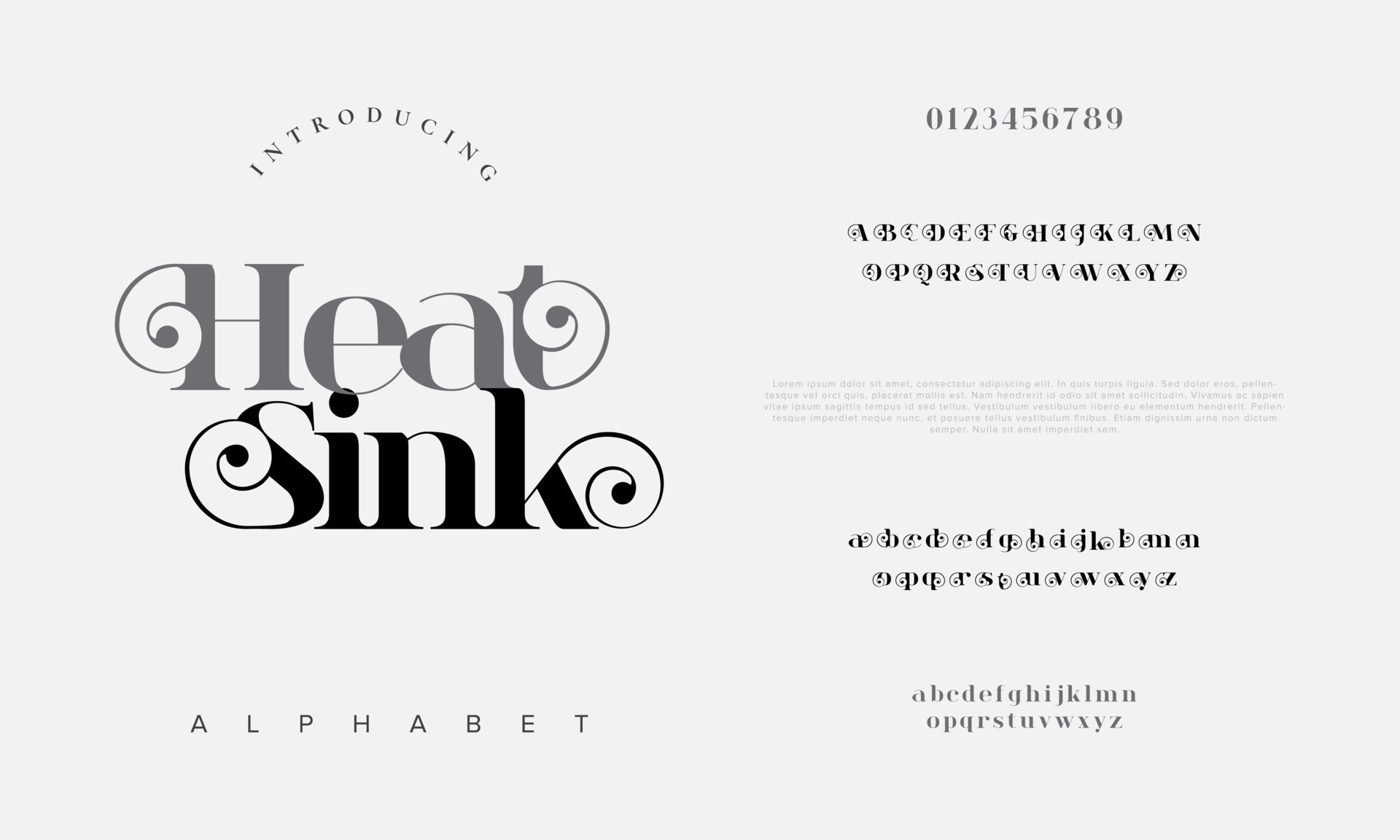A detailed and descriptive caption for the image could be:

---

This poster showcases the introduction of a new typeface designed for typography enthusiasts. On the left-hand side, the word "Introducing" is prominently displayed in a semi-circle, all in capital letters, drawing immediate attention. The typeface is aptly named "Heat Sink," and just below the title, there is another text that reads "Alphabet." 

On the right-hand side, the poster features a collection of visually striking capital letters, each exuding an ornate flair with intricate swirl embellishments. A sequence of numbers complements the elaborate letterforms. Additionally, there is some partially obscured text in a faded grey tone, lending an air of mystery and depth to the design. The entire color scheme of the poster is a sophisticated blend of grey, white, and black, creating a monochromatic yet dynamic visual experience.

Below the ornate capital letters, the typeface continues with a set of lowercase letters, each also adorned with delicate swirlies, maintaining the cohesive decorative style. At the very bottom of the poster, a greyed-out section displays a more straightforward lowercase alphabet without the ornamental details, providing a clean contrast to the rest of the typeface.

---

This caption elaborates on the original description, providing a clear and detailed narrative of the poster's content and design elements.